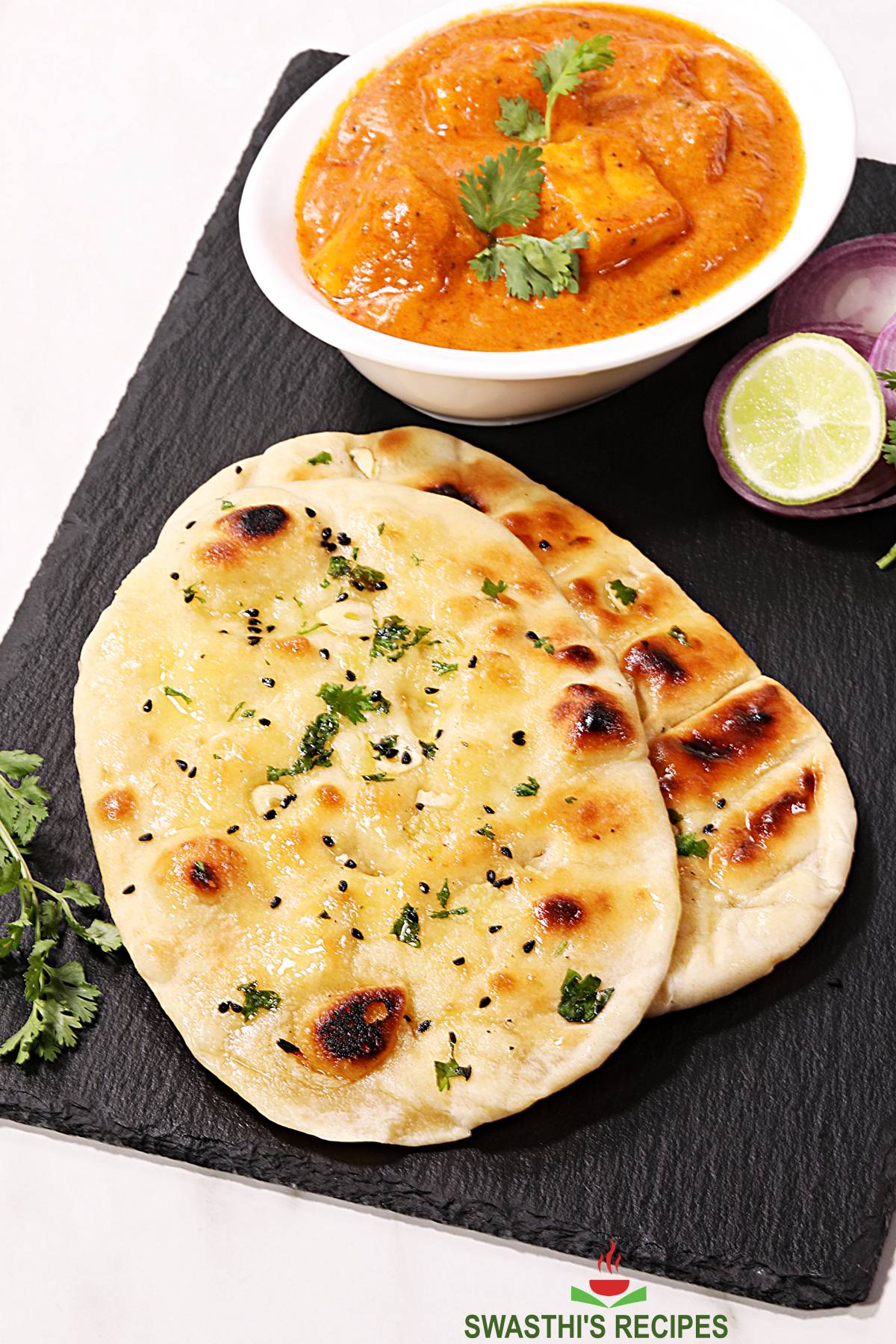The photograph features a vibrant and appetizing food arrangement displayed on a rectangular black slate platter. In the foreground, there are two pieces of grilled naan bread, slightly charred to perfection, sprinkled with green herbs and overlapping each other. A sprig of fresh parsley lies nearby as a garnish. Centered on the platter is a small, white bowl containing an orange-hued stew, which appears to feature chunky pieces of meat or tofu and is topped with more parsley. Just to the right of the bowl, there are slices of lemon and onion. The entire setup is visually striking with its bright colors, enhanced by the black background of the slate. The words "Swathees Recipes," alongside a small red and green logo, are visible at the bottom of the picture, adding a personalized touch to the presentation.